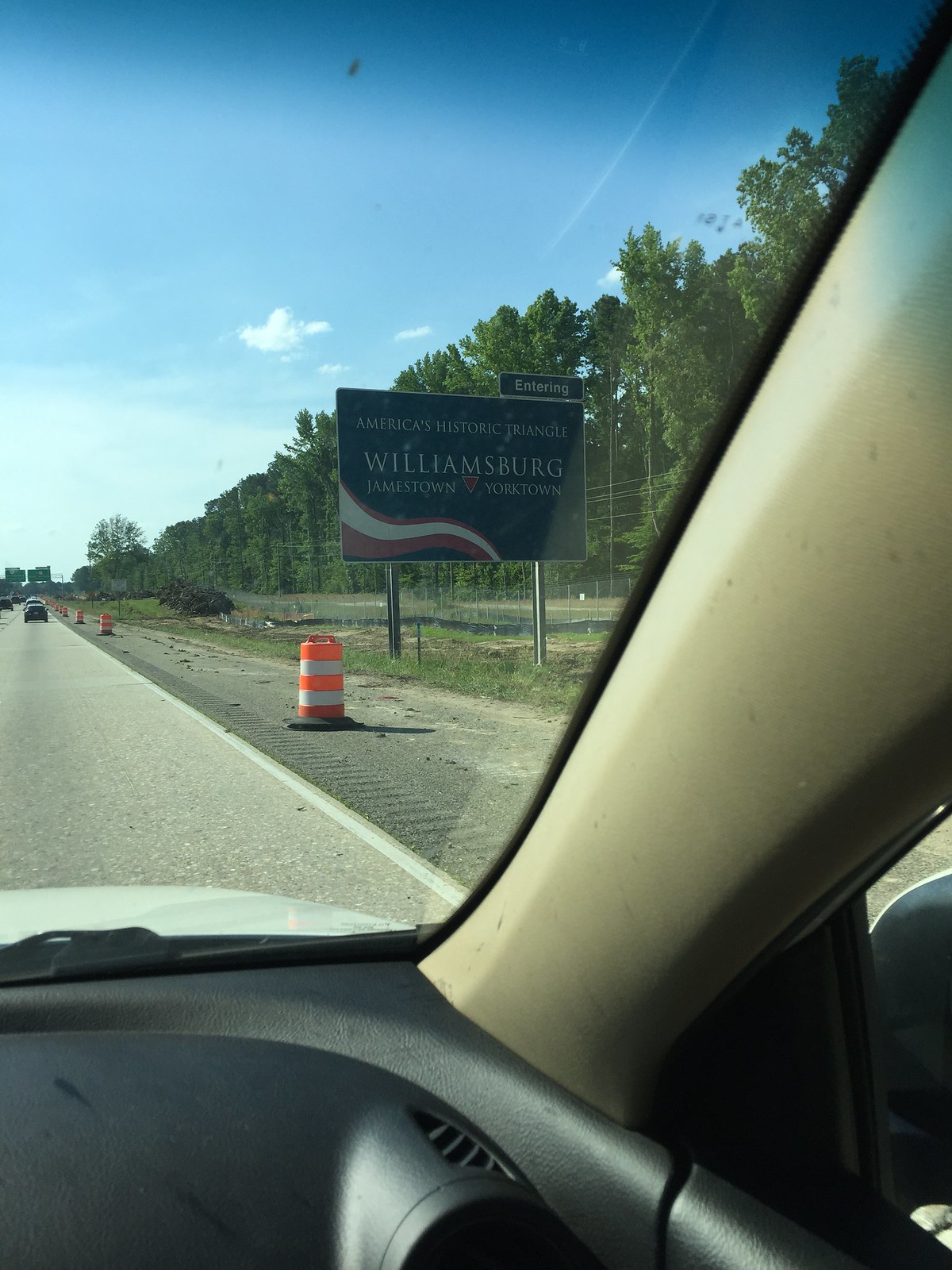This photograph, taken from the passenger seat of a car, captures a clear view of a highway lined with traffic cones featuring white and orange stripes. Prominently positioned on the right-hand side of the road is a striking sign with a red and white swirl at the bottom, announcing the entrance to "America's Historic Triangle: Williamsburg, Jamestown, Yorktown." The sign features gold and red elements and is part of a tree-lined landscape under a blue sky dotted with fluffy clouds. The foreground of the image includes glimpses of the car's interior, revealing a portion of the black dashboard, a vent, and part of the passenger side window. The highway itself is relatively free of traffic, with only a few cars visible further down the road, and the presence of road rivets, which vibrate cars that drift over them, adds further detail to the scene.